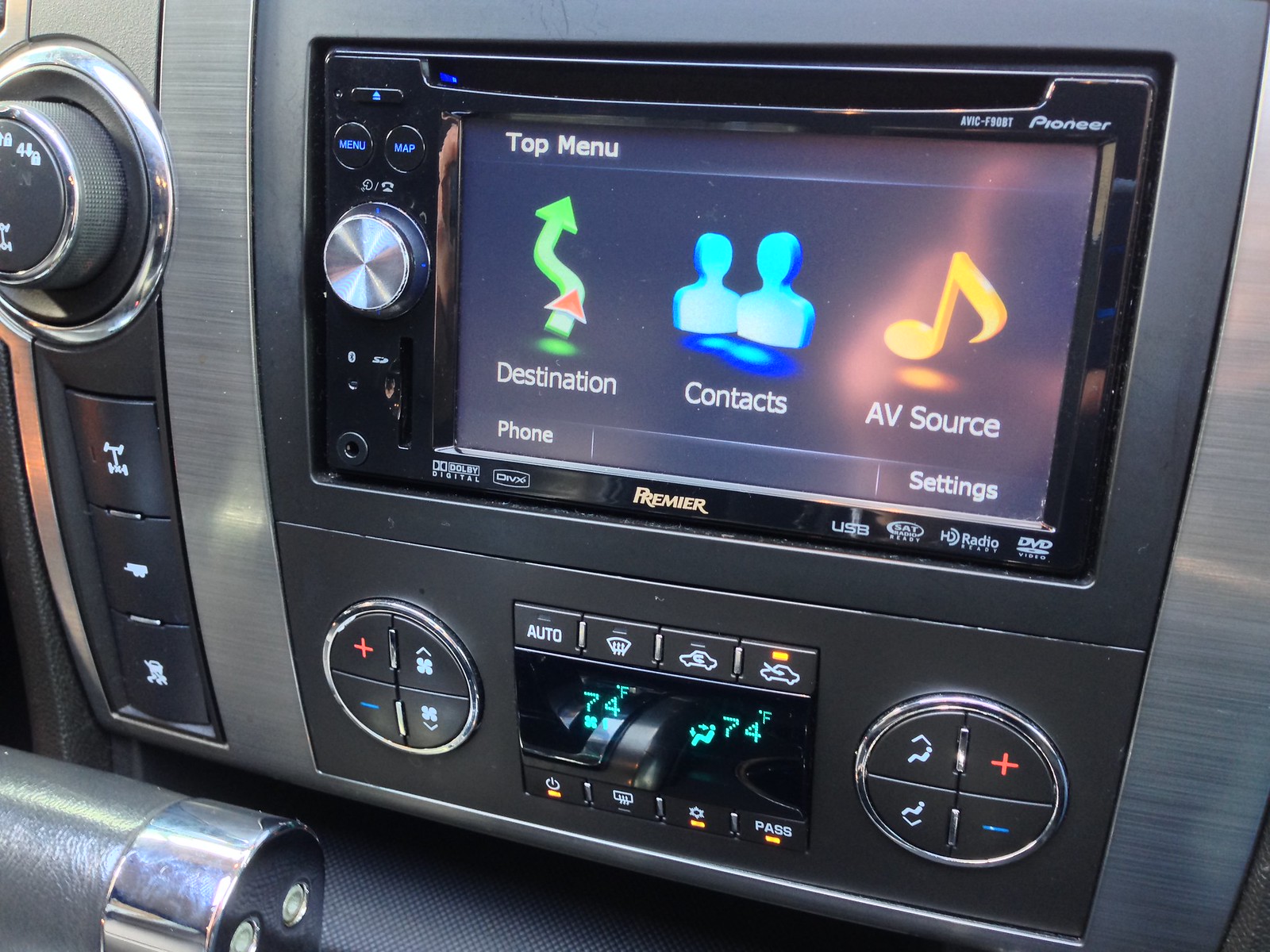The image is a full-color photograph taken inside a car during the daytime, without a border. The focus is on the gray-hued interior of the vehicle, specifically a close-up of the dashboard's central console. The dashboard showcases a digital display screen positioned centrally and slightly tilted from left to right. On the screen, it reads "Top Menu" and lists various options such as "Destination" with an arrow, "Contacts" represented by silhouettes, "AV Source" with a musical note, "Phone," and "Settings." Above the display, it shows "Pioneer" and the current temperature in the car, which is 74 degrees. Below the screen, there are numerous buttons and knobs for controlling the car's functions, including traction control, air conditioning, circulation, and window defroster. The fan and seat control buttons are clearly marked with plus and minus signs. The dashboard's color scheme comprises various tones: orange, bright green, bright blue, shades of gray, black, and faded metallic hues. The overall setup indicates a well-equipped, modern vehicle with an emphasis on user control and comfort.